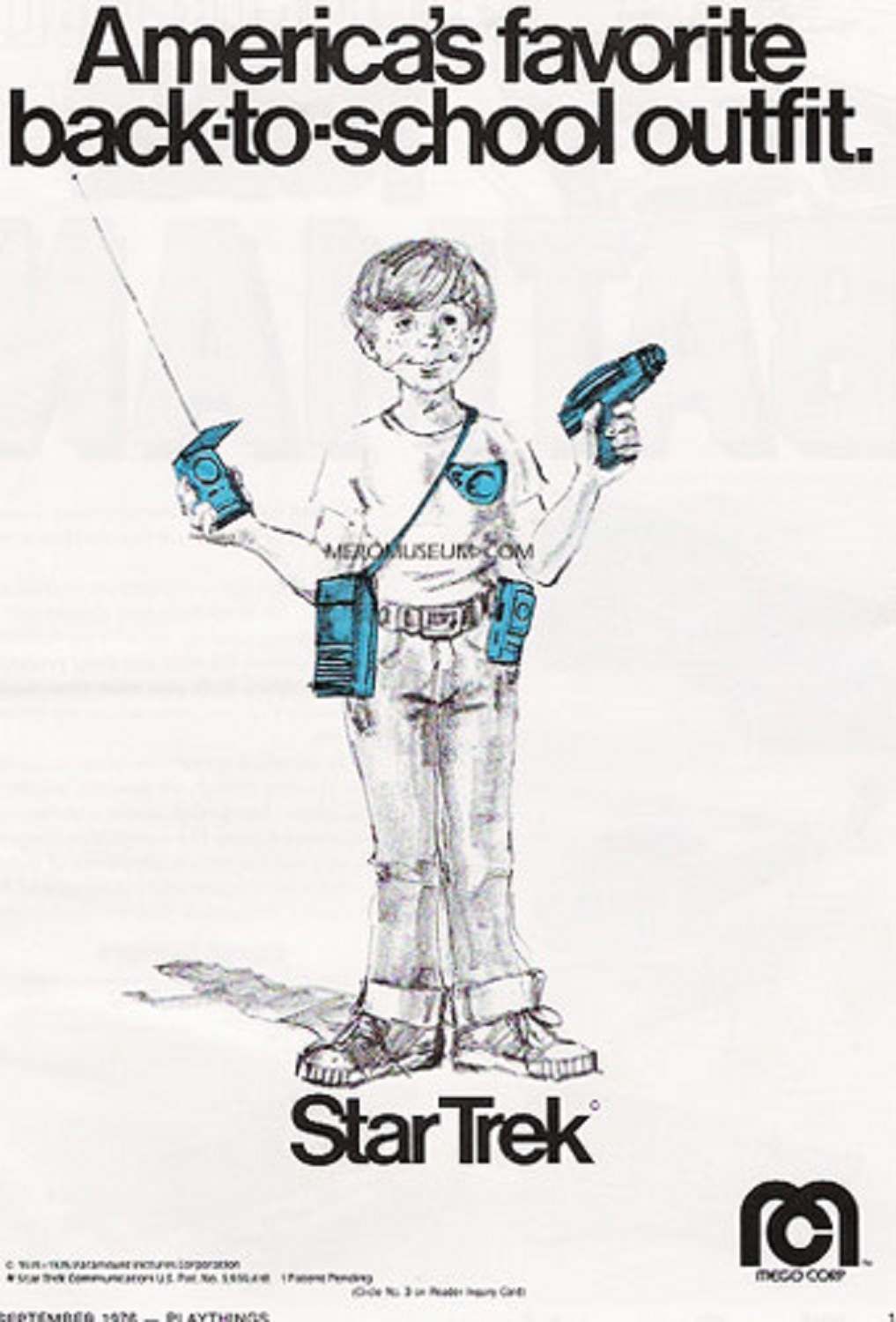The image is an advertisement predominantly in black and white with touches of blue, featuring text at the top that reads, "America's Favorite Back-to-School Outfit." Below this text is a detailed drawing of a boy, possibly around 10 years old, dressed in a retro back-to-school ensemble. He wears rolled-up jeans and tennis shoes, and his T-shirt is tucked in. Distinctively, he sports a mix of accessories that evoke a Star Trek theme. In his left hand, he holds a blue ray gun or phaser, and in his right hand, he carries a blue tricorder or remote control. Attached to his belt are various gadgets, including what appears to be a walkie-talkie and another similar device, also accented in blue. He has a badge on his shirt and a blue shoulder bag. The boy's cheerful face is highlighted with freckles. Beneath the illustration, the text "Star Trek" is prominently displayed in black letters. In the bottom right corner of the ad, a logo reads "Mego Corp," accompanied by an "MC" emblem and the number "1," possibly indicating the first page of a magazine. Although the smaller text towards the bottom is difficult to decipher, it further cements the nostalgic feel of this 1960s or 70s advertisement.